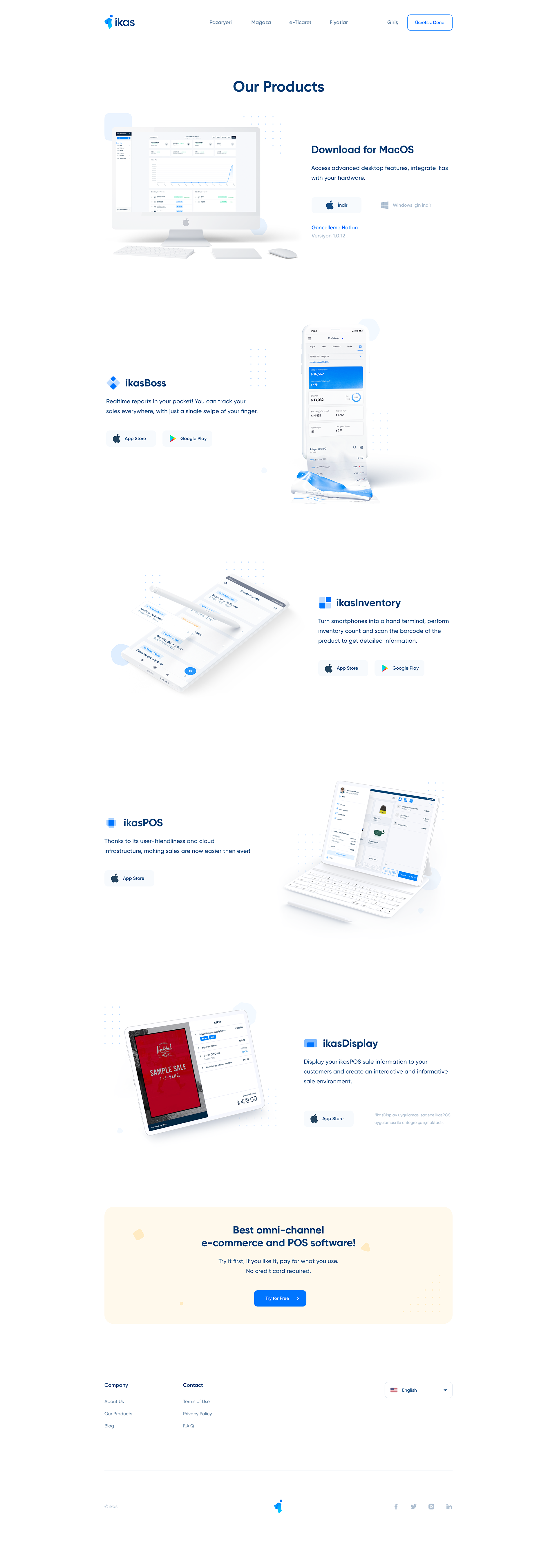The image depicts a long, scrolling webpage with a white background, showcasing various products under the header "Our Products." In the upper left corner, the "ICAS" logo, which resembles a blue arrow, is visible. At the top of the page, there is a computer displaying graphs and the text "Download for macOS."

As you scroll down, the webpage details several applications. "ICAS BOSS" is shown running on a smartphone. Below that, "ICAS Inventory" is listed, followed by "ICAS POS," which is displayed on a laptop. Further down, "ICAS Display" is featured on a dual-display device, running ICAS software.

At the bottom of the page, bold text proclaims, "Best Omni-channel e-commerce and POS software." The page also features small-font text options for language settings. Each product section has its own header and description, aligning with the clean, white background.